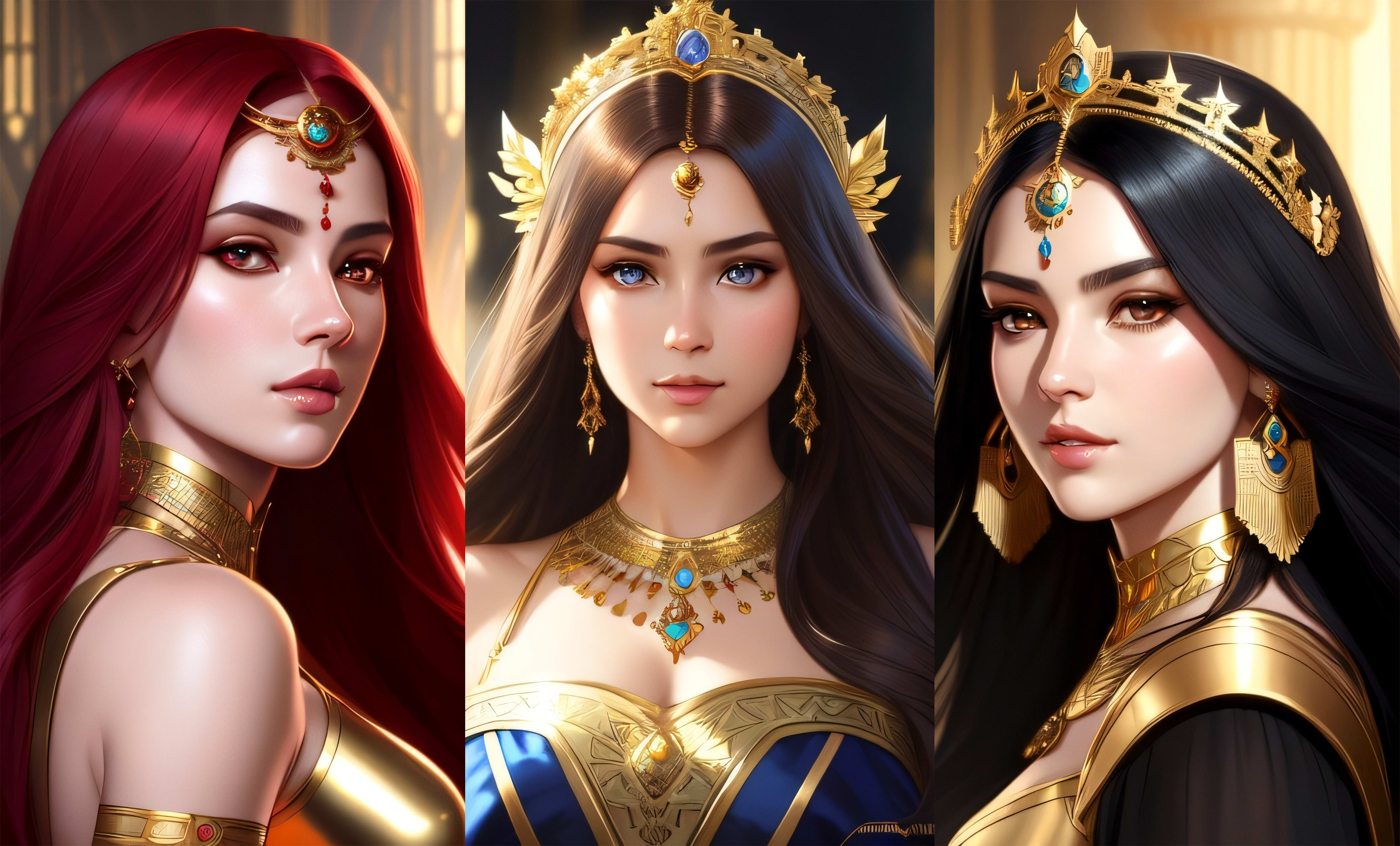The rectangular composite image comprises three distinct digital artwork pieces, each depicting a different woman, arranged vertically. All three women share certain thematic elements like crowns and gold attire, but each has unique features. The artwork has a sleek, glossy style suggestive of AI-generated visuals.

The leftmost woman faces right but looks directly ahead, showcasing bright red eyes and long dark red hair that falls past her shoulders. She adorns a gold collar around her neck and a dangling gold crown on her head. Complementing her regal look is a form-fitting, sleeveless gold chest plate cut off at the shoulders.

In the center, the woman wears a luxurious blue and gold dress with a low neckline that reveals a hint of cleavage. Her accessories include a gold necklace with a blue pendant, matching the hue of her blue eyes. Atop her head is a gold crown, and she has hazel brown hair cascading down.

The rightmost artwork presents another distinct woman with black hair and hazel eyes, wearing a stylish gold dress. She features a gold crown similar to the center figure but slightly varied in design. Her look is completed with blue and gold dangling earrings that catch the light, adding a touch of elegance to her appearance.

The overall image portrays an intriguing mixture of similarity and individuality among the women, unified by the ornate golden motifs and contrasting colors.